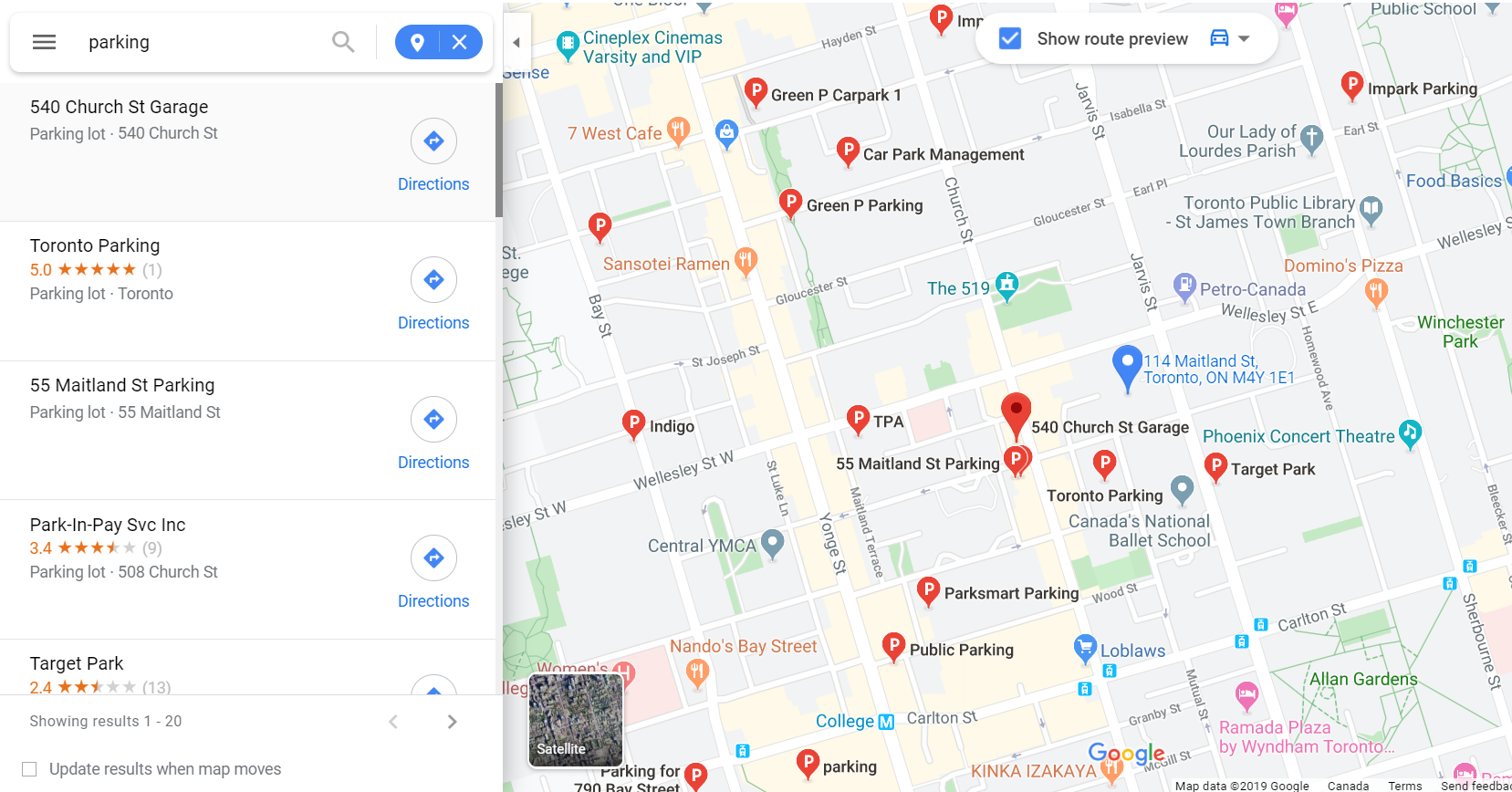**Detailed Image Caption:**

The image depicts a detailed map of Toronto, Canada, highlighting various notable locations and facilities. At the center of the map, a prominent green pin marks the location of Cineplex Cinemas Varsity and VIP, surrounded by an array of diverse restaurants and eateries. The map is dense with multiple blue parking markers indicating the abundance of public parking options available throughout the area.

On the left side of the image, there is a search bar. To the left of the search bar is a hamburger menu icon, which provides additional options when clicked. The map is currently displaying search results for parking, identifiable by the specific pins, which users can choose to show or hide. Below the search bar, a list of parking facilities is displayed, offering detailed information and navigation options for each.

The first entry on the list is the "540 Church Street Garage," located at 540 Church Street. Users can easily get directions to this garage. Next on the list is "Toronto Parking," which boasts a stellar five-star rating, indicating it is a highly favored parking lot in the city. Following this is "55 Maitland Street Parking," a parking facility situated at 55 Maitland Street, with navigation options available.

Further down the list is "Park and Pay SVC Incorporated," which has a moderate rating of 3.4 stars based on nine reviews. There is also another entry for "Toronto Parking with a singular rating, marking its importance. Close by is a parking lot at 508 Church Street, maintaining close proximity to the previously mentioned garages.

Lastly, the list includes "Target Park," which holds a lower rating of 2.4 stars out of five, suggesting it may not be the preferred choice for many users. This extensive listing provides an insightful guide to parking in Toronto, helping users find the best options suited to their needs.